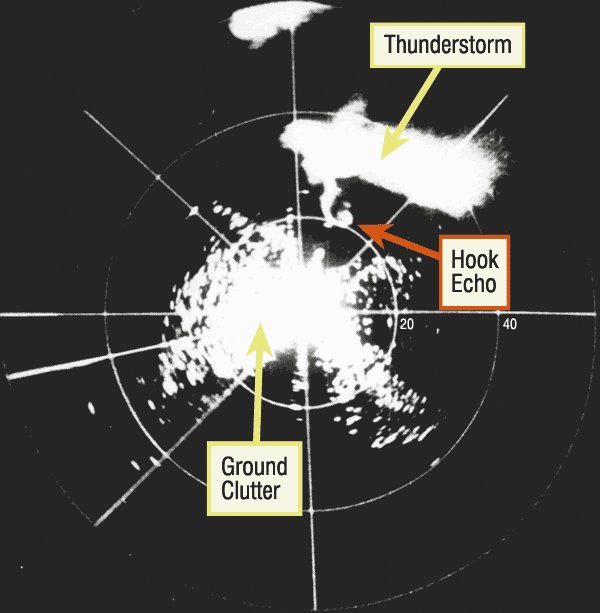The image depicts a digitally created, weather tracking diagram centered on a black square. A prominent white bullseye with various colored splatters marks the middle, dissected by circles and lines pointing in multiple directions. The diagram includes labels and arrows to indicate specific weather phenomena: "thunderstorm" is highlighted in an orange-yellow box positioned in the top right, "hook echo" in an orange box in the middle right center, and "ground clutter" in a yellow box at the bottom left. Additional numerical markers, such as 0-20-40, are present around the bullseye. The visual composition features a palette of red, yellow, white, black, and off-white, establishing a comprehensive storm tracking representation. Notes like "Go to Beadaholique.com for all of your beading supply needs!" appear extraneously.